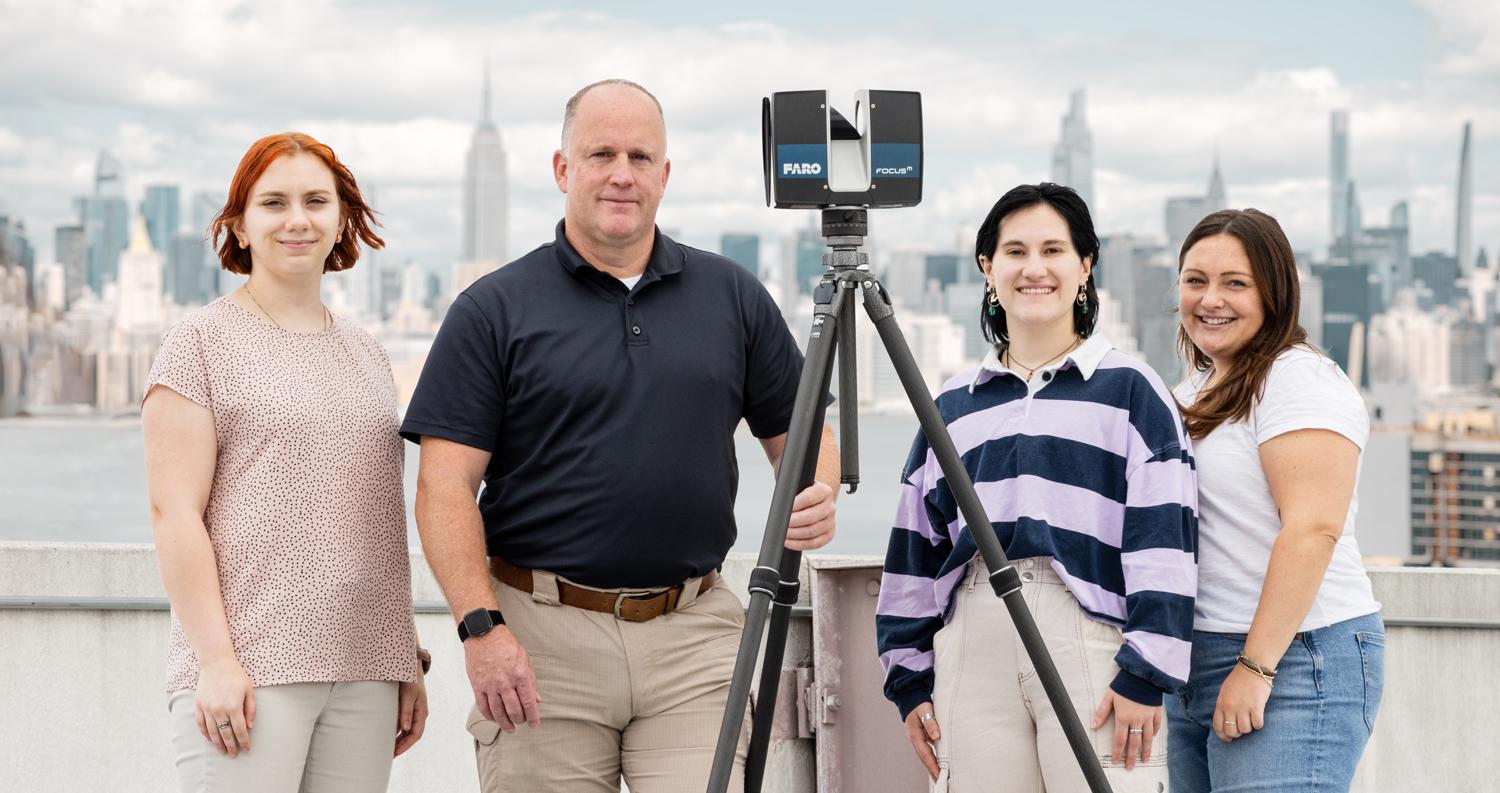In this detailed photograph, four individuals stand on a rooftop against the backdrop of a somewhat blurred, yet recognizable city skyline, possibly New York, under a blue sky speckled with clouds. Central to the image is a tripod topped with a device labeled "FARO," though its exact function—be it a camera or stabilizer—remains unclear.

To the left stands a woman with shoulder-length red hair, wearing a pink blouse with dark purple polka dots and white pants. She appears younger, perhaps in her mid-20s, and on the chubby side. Next to her, a middle-aged man, possibly in his late 40s to early 50s, dons a black polo shirt, khakis with a brown belt, and a black digital smartwatch. He appears professional and holds onto the tripod, enhancing the image’s focal point.

On the right, a pair of women, also seemingly in their mid-20s, share the space. Closest to the man is a woman with long dark hair, adorned with earrings, dressed in a purple and blue striped shirt and khaki pants. Beside her stands another woman with medium-length brown hair, smiling, in a simple white t-shirt and blue jeans.

Together, they appear either as a family or close-knit group. The device on the tripod potentially offers a way to zoom in on the urban landscape behind them, adding an intriguing element to their pose.